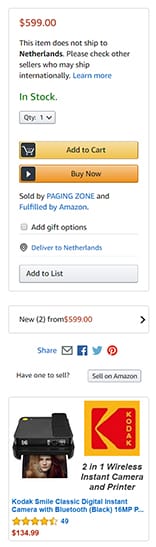This image is a stretched screenshot of the bottom section of an Amazon.com mobile product purchasing page, focusing on the price and select options. At the top, the price is prominently displayed in red as $5.99. Below the price, there is a message indicating that the item does not ship to the Netherlands, with a suggestion to check other sellers for international shipping options. A small blue "Learn more" link follows this message.

In bold green text, the availability status is shown as "In Stock", and below this, there is a drop-down box set to a quantity of one. Beneath the quantity selector, there are two buttons: a yellow "Add to Cart" button and an orange "Buy Now" button.

The item is sold by "Paging Zone", with both the seller's name and "Fulfilled by Amazon" hyperlinked in blue. Additional options are provided, such as "Add gift options" and a hyperlink stating "Delivered to the Netherlands". Another option "Add to List" is also available.

Towards the bottom of the page, there are sharing options via email, Facebook, Twitter, and Pinterest. Finally, there is a prompt that reads "Have one to sell? Sell on Amazon."